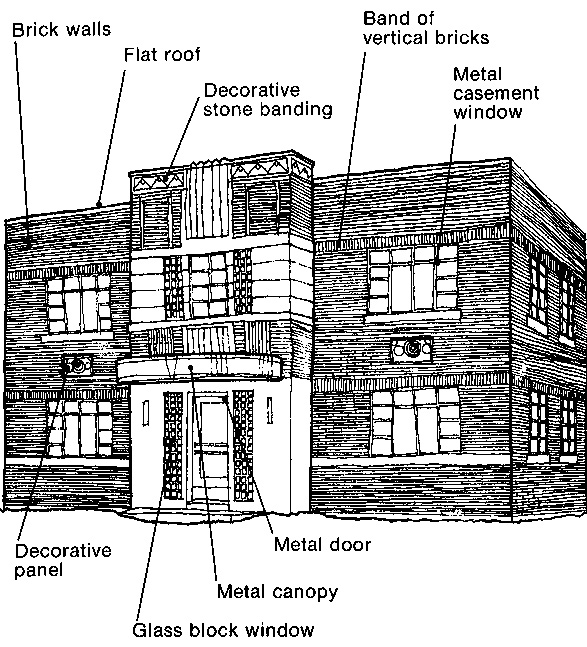This is a black and white 3D pencil drawing of a two-story brick building, meticulously labeled to identify various architectural features. The illustration includes detailed lines pointing to specific parts of the building, with corresponding labels such as "brick walls," "flat roof," "decorative stone banding," "band of vertical bricks," "metal casement windows," "metal door," "metal canopy," "glass block window," and "decorative panel." The drawing likely resembles an architectural illustration, possibly featured in a book. The entryway is distinct, slightly protruding from the main structure, and is highlighted with white brick and flanked by glass block windows. The building, which appears to be designed for public use such as a theater or event venue, features a total of eight windows—four on the front and four on the side. The precise and informative nature of the drawing gives an insightful view into the building's design without any additional authorial or temporal context.